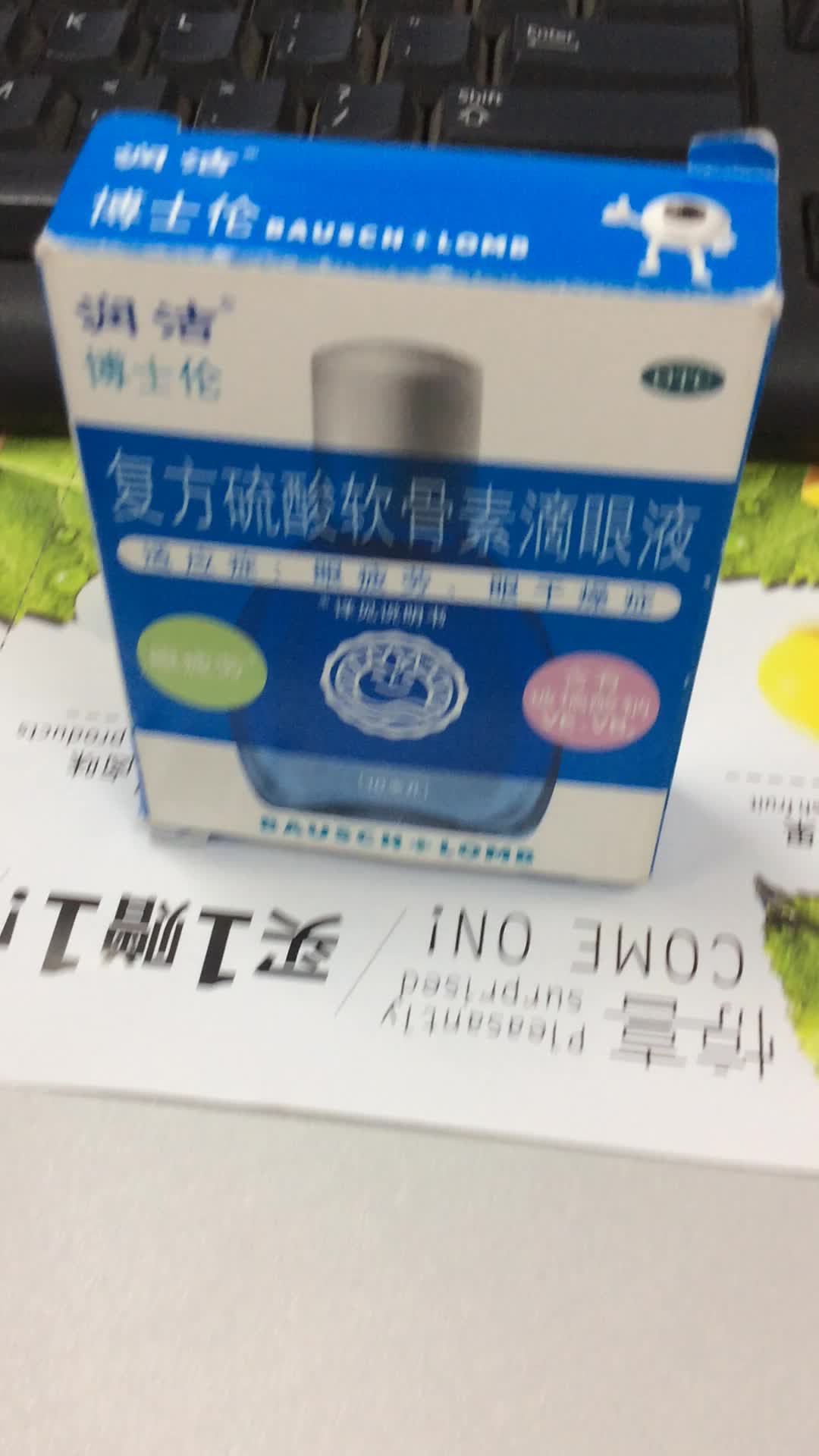The image depicts a blurry photograph of a box standing upright on a light gray surface, partially obscuring some upside-down white papers with visible but unreadable Japanse or possibly Chinese characters. The box has a blue top featuring white writing and an animal illustration on the right side. The front face of the box is predominantly white and blue, displaying a blue-tinted bottle with a white cap, although most of the bottle is obscured by a blue label with white Asian characters. Below the bottle image, there's a strip of white with blue text, followed by three round emblems. In the background, out of focus, a computer keyboard and a poster with the phrase "come on" can be faintly seen.